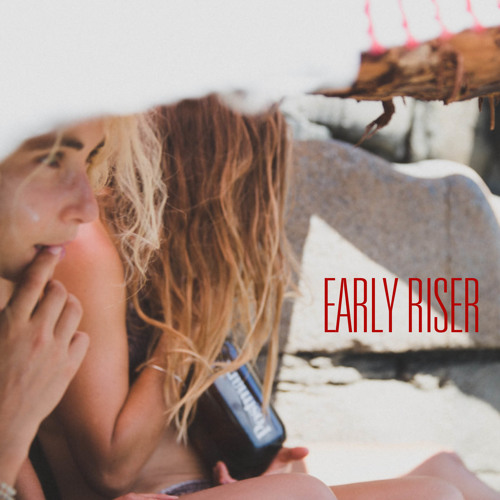The image appears to be an abstract and possibly stylized album cover set in an outdoor setting reminiscent of a beach, featuring two individuals. The first person, situated on the left, is likely a man with a curious expression, holding his forefinger to his mouth as he gazes into the distance. The second person, positioned to the right, is a woman with long, streaky brownish-blonde hair partially obscuring her face. She seems to be holding a black bottle, possibly a liquor bottle. They are both wearing beach attire; she is donned in a bikini, while the man's outfit is less discernible.

The setting features a number of distinct elements, including a rock-like structure or sculpture in the background, which is somewhat out of focus and obscured. A wooden post or log is visible in the upper corners of the image, adding to the beach-like atmosphere. The overall scene is framed in such a way that parts of their bodies, particularly their faces, are not fully visible, lending a mysterious and abstract quality to the photograph.

Red text reading "Early Riser" is positioned off to the right side of the image, suggesting this may indeed be an album cover. The combination of the beach setting, the rock structure, and the positioning of the individuals creates a compelling and enigmatic visual narrative.